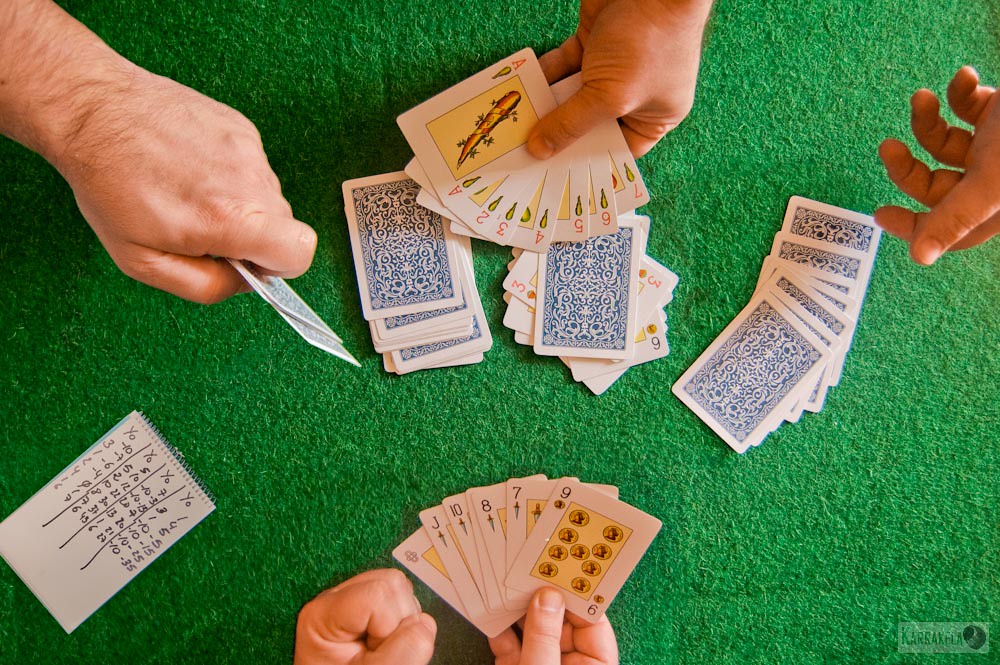In this horizontal, landscape-oriented image, a group of individuals is engaged in a game of cards on a green, carpeted table, likely a pool table. The photo is captured from a first-person point of view, reminiscent of a GoPro angle. The foreground depicts two hands at the bottom: the left hand is clenched, and the right hand fans out a hand of cards. The visible cards include a nine with nine yellow-circled pips on a white-bordered, yellow background, followed by a seven, eight, ten, Jack, and an obscured card. To the left of this central figure lies a handwritten scoreboard with multiple columns. On the upper left, a man's hand holds two cards, while at the top of the image, another player's hand grips several cards. Scattered face-down cards are visible across the table, and on the right side, another open hand can be seen, indicating a dynamic and engaging card game in progress.